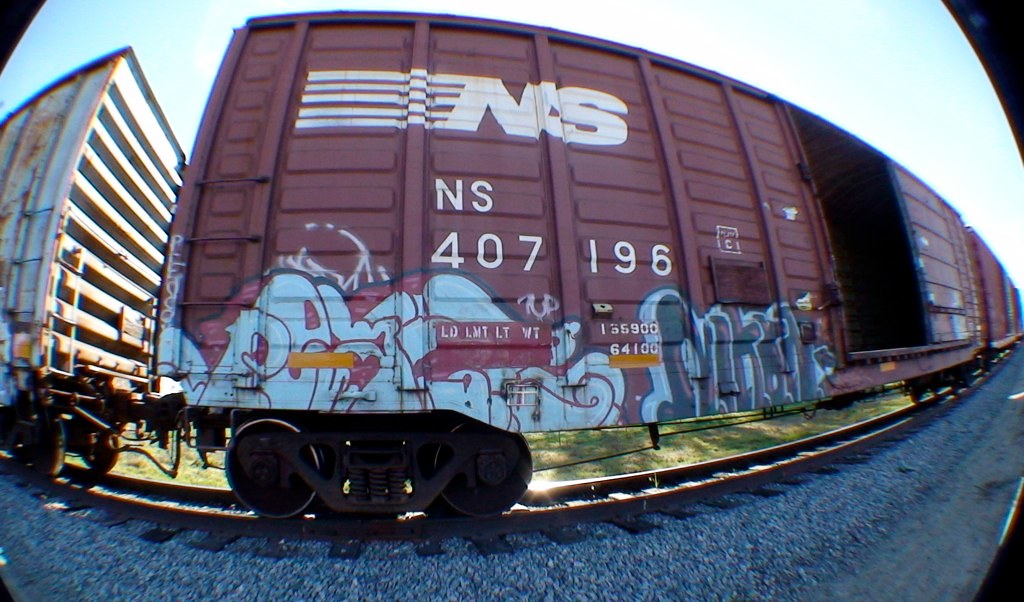The photograph showcases a distorted, fisheye lens view of a dark purple-burgundy freight train car on a set of curved tracks, during the day under a bright blue sky. The centerpiece of the image is a close-up of this particular car, which prominently features the initials "NS" at the top left-hand corner, followed by "NS407196" beneath it. The car is adorned with graffiti along its lower section, displaying a mix of light blue and slate gray colors, with some designs resembling ghostly faces with grimaces, though the exact lettering is illegible. Additionally, there are technical markings including "LD LM TLT WT" and numbers "135900 64100." The car also has an open door, revealing an empty interior, and is connected to a white train car behind it, with another red car visible at the front. The surrounding area consists of gray gravel tracks and a patch of green grass.